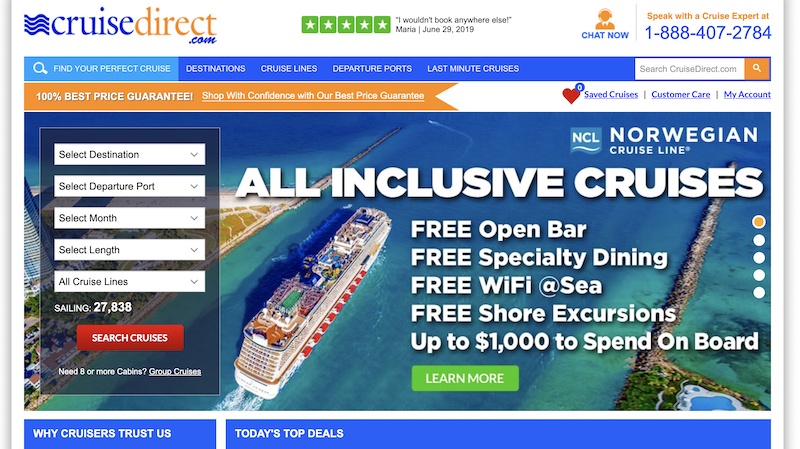**Detailed Caption:**

The image is a desktop screenshot of a website, specifically CruiseDirect.com. The logo is located at the top left corner, featuring the word "Cruise" in blue letters, "Direct" in orange letters, and "dot com" again in blue letters. At the top middle portion of the screen, there is a five out of five stars review, represented by green squares each containing a star. To the immediate right of the review, it states, "I wouldn't book anywhere else," attributed to Maria with the date June 29, 2019. Further to the right, there is a "Chat Now" option, and next to it, the text reads "Speak with a cruise expert at 1-888-407-2784."

Beneath this header section, there is a functional magnifying glass (search icon) within a search bar that prompts users to "Find Your Perfect Cruise." To the right of this search bar are four tabs, each on a blue background: "Destinations," "Cruise Lines," "Departure Ports," and "Last Minute Cruises." Adjacent to these tabs is a white input field marked "Search CruiseDirect.com" with another magnifying glass icon.

Below this, the site highlights its "100% Best Price Guarantee," encouraging visitors to shop with confidence. Adjacent to this phrase, a red heart icon pairs with the words "Safety and Cruises." Moving rightward, there are clickable options for "Customer Care" and "My Account."

Dominating the central part of the screenshot is an image of a cruise ship sailing towards the horizon. Above the ship image, the text advertises "All-Inclusive Cruises by the Norwegian Cruise Line (NCL)." Below this header, several offers are listed: "Free Open Bar," "Free Specialty Dining," "Free Wi-Fi at Sea," "Free Shore Excursions," and up to "$1,000 to Spend Onboard." Just beneath these benefits, there is a green rectangular "Learn More" button.

This detailed layout underscores the site's focus on providing a comprehensive and enticing cruise booking experience.